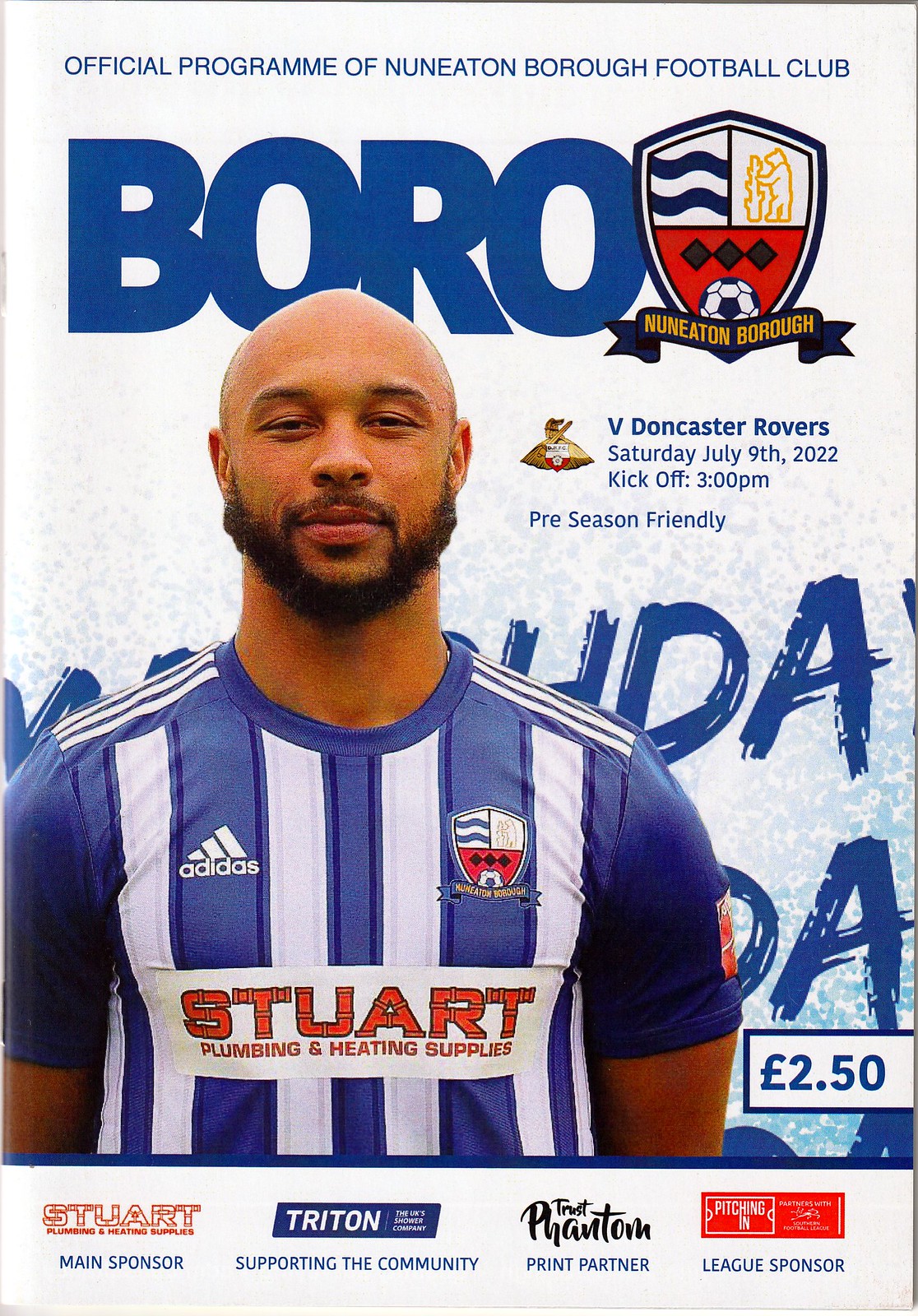This magazine cover features a predominantly white background with striking blue and orange elements. At the top, bold uppercase letters in solid blue spell out "BORO" on the left. Adjacent to that, on the right, is a shield and emblem indicating "Newton Eaton Borough" in orange and blue. 

The primary focus of the cover is a color photograph of a soccer player, shown from the chest up, dressed in a blue jersey with white stripes. Emblazoned on his chest is the text "Stewart Plumbing and Heating Supplies" in orange, with the Newton Eaton Borough logo also visible on his upper chest. Behind the player, indistinct blue text is present, with only the letters "D" and "A" repeating.

To the right of the player’s head, blue text announces a match: "V Doncaster Rovers," scheduled for Saturday, July 9th, 2022, with a kickoff at 3 p.m., marking it as a preseason friendly. The magazine is priced at £2.50.